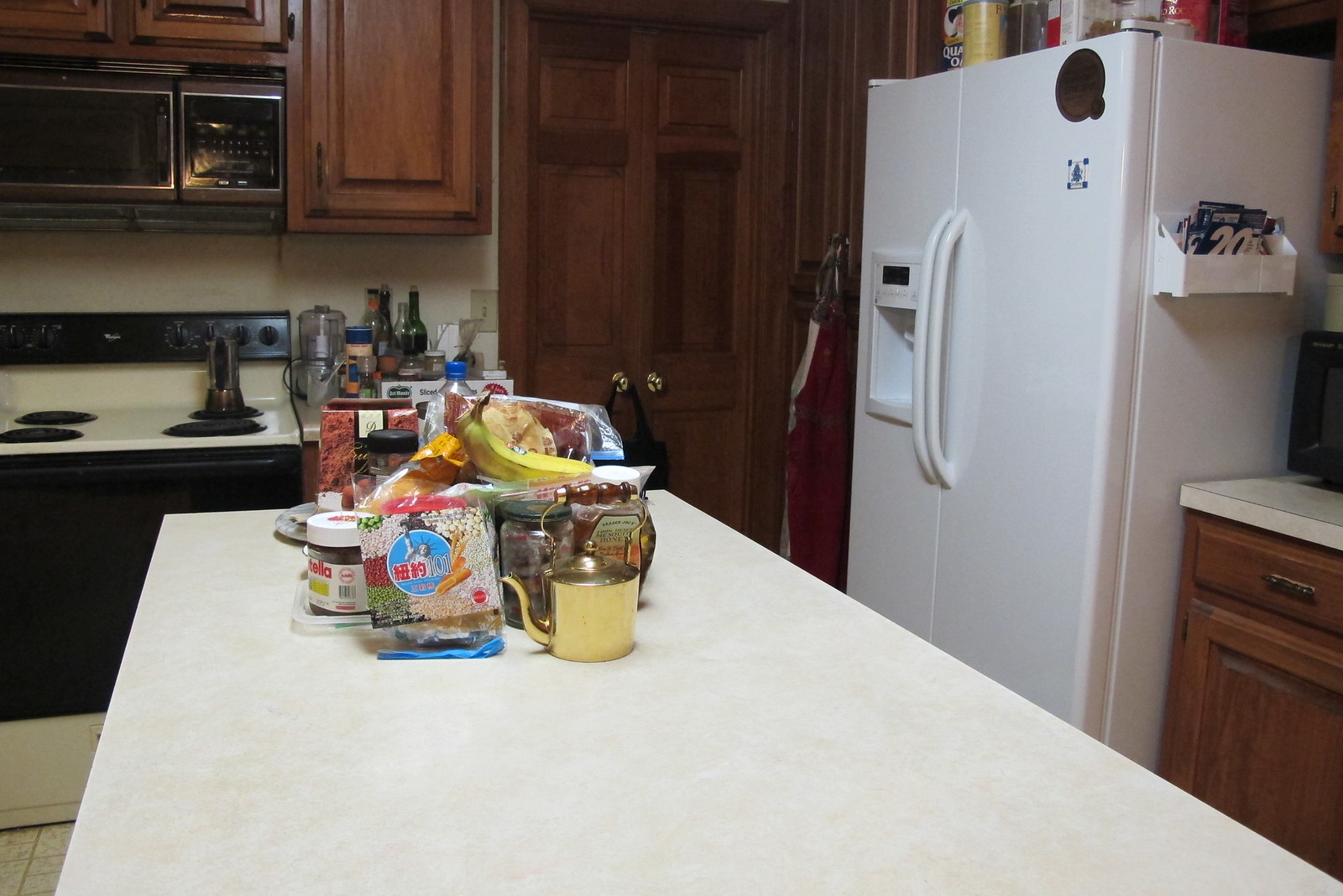In the photograph, a quaint kitchen scene is depicted, showcasing a central plain white countertop island that acts as the focal point of the image. At the far side of this island, various food items are grouped together. To the right of the scene stands a white refrigerator, flanked by several cupboards featuring an older wood style on both left and right sides.

On the left, beneath the cupboards, there is a microwave and a stove. Additionally, a closed wooden door hints at either a pantry or a small closet. Adjacent to the refrigerator, a wooden pantry or small closet, and a bottom drawer are visible.

The food assortment on the island includes a prominent gold tea kettle positioned at the front right. To the left of the kettle, an indistinct item is partially visible. Slightly behind the kettle stands a jar of Nutella, flanked by bananas on the right. Also on the right side, there’s a Ziploc bag, while on the left side, a partially visible item with a red label adds to the assortment. The kitchen exudes a homely, functional ambiance with its combination of modern and rustic elements.